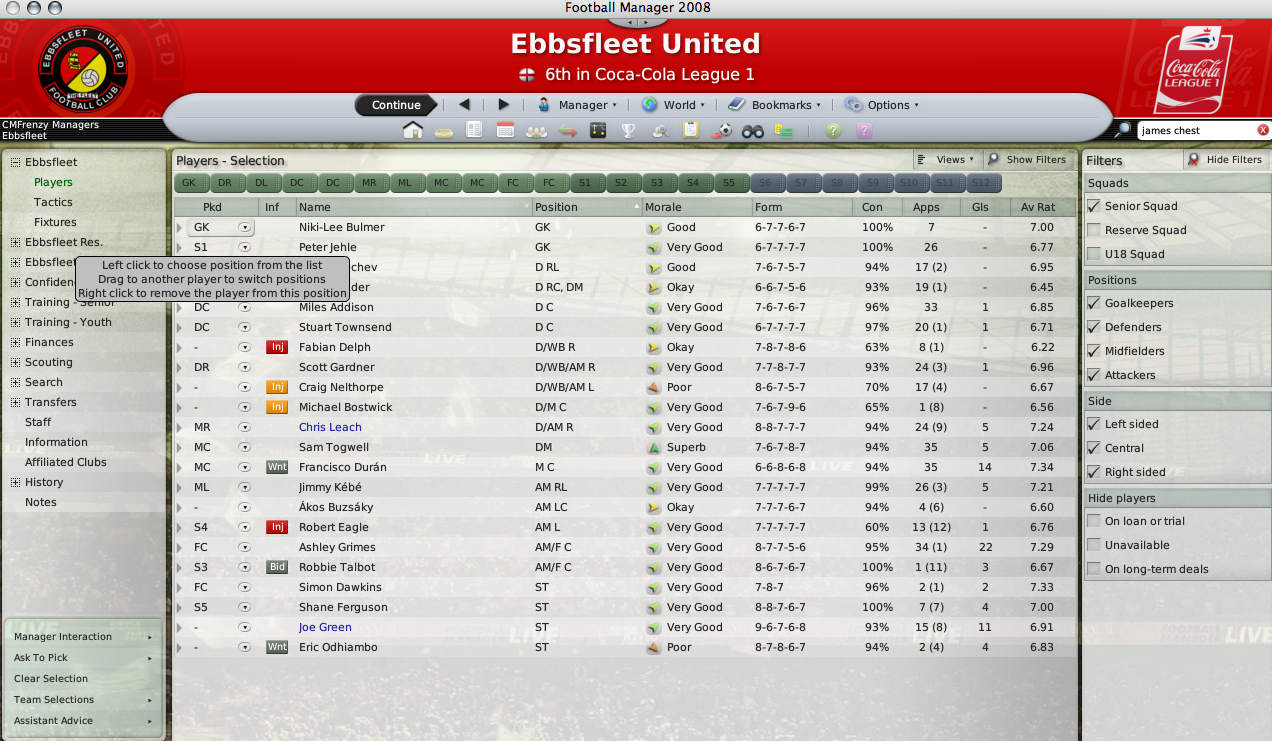This image is a detailed screenshot of the Football Manager 2008 application running on an older version of Mac OS, distinguished by the characteristic three buttons on the top left of the title bar. The title bar clearly reads "Football Manager 2008," and just below it, in a prominent red banner, it states "EBS Fleet United, sixth in Coca-Cola League One," flanked by the club's emblem on the left and a Coca-Cola sponsorship emblem featuring a football symbol on the right. The interface showcases a highly interactive and user-friendly layout designed for managing and analyzing team data.

At the center of the image, a comprehensive data table is titled "Players Selection," displaying detailed statistics across approximately nine columns, set against a light gray background. Below the banner, an elongated, rounded rectangular menu offers various clickable options and tools such as manager, world, bookmarks, and options buttons, accompanied by icons representing a house, an ashtray, newspaper, calendar, and more, suggesting diverse functionalities.

On the left side of the main body lies a collapsible, tree-style menu that lists different teams or managers, including the Ebbs Fleet United Club's senior squad, indicated by a checkbox with a checkmark. The right side of the interface contains additional interactive elements, such as a search bar, squads menu, positions menu, and filters menu, each accompanied by checkboxes for customized data viewing.

In summary, the screenshot presents an advanced, multifaceted statistical resource specifically for the Ebbs Fleet United Football Club within the Football Manager 2008 game, reflecting its practical utility for fans, coaches, and players.